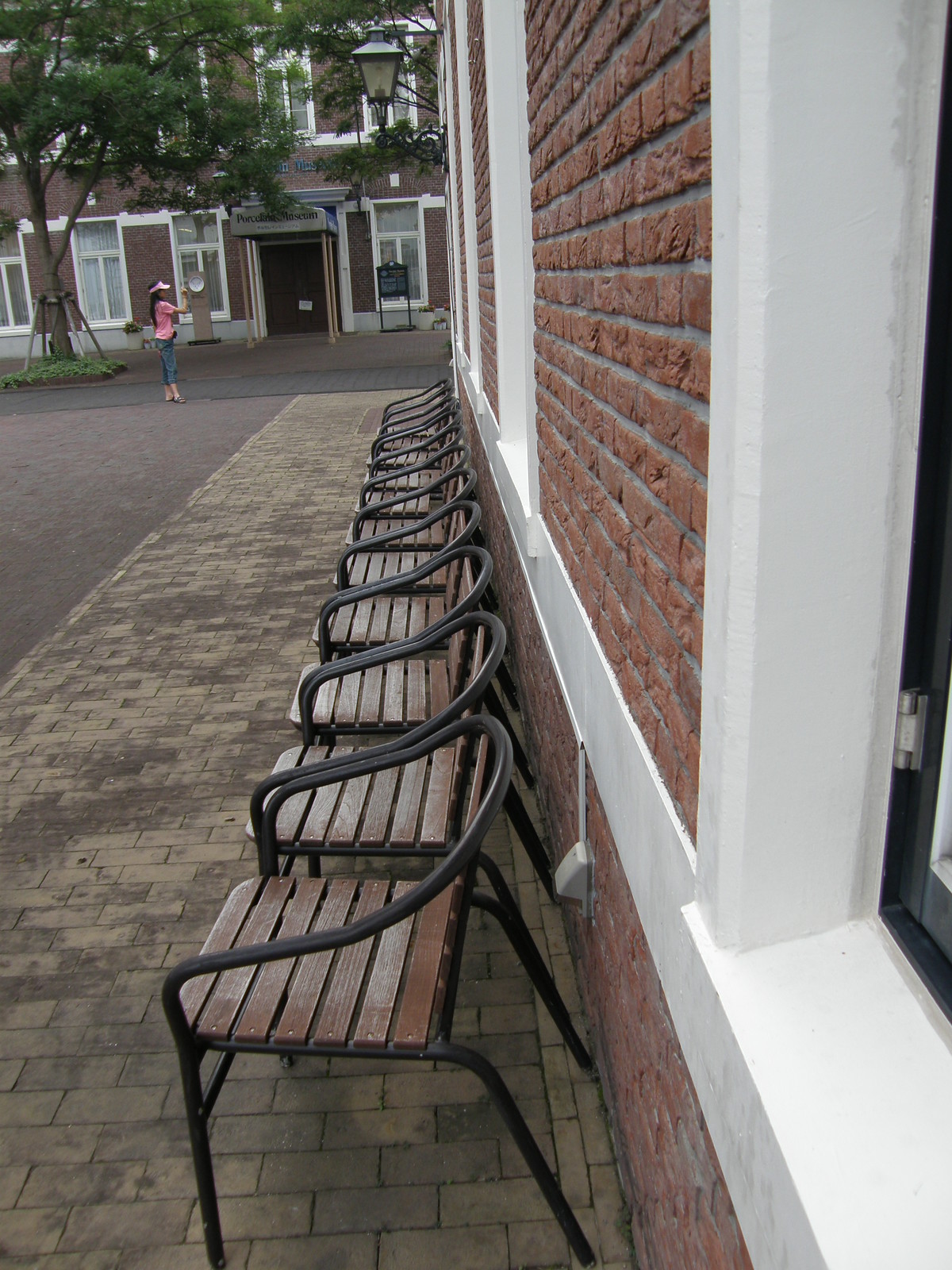This photograph captures a historic architectural scene centered around a red brick building with white trim, featuring three to four large black-framed windows. In front of this building, a row of approximately ten wooden slat chairs, with black metal legs and open backs, is neatly aligned on a cobblestone sidewalk of light brown bricks. The chairs, side-facing the camera, exhibit a distinct contrast with their dark wooden seats and black iron framework against the deep red brick wall. 

To the right edge of the photograph, a black plaque, likely indicating the building's historical significance, is visible. The background reveals another red brick structure with similar white trim and several windows, adding depth to the scene. A paved street of maroon bricks runs parallel to the sidewalk, transitioning into a more traditional dark gray paved area. 

In the upper left corner, a woman with long black hair is present, dressed in a pink t-shirt, blue capri jeans, and a pink visor. She appears to be taking a photograph, possibly of the historical site, near a small tree housed in a planter. The setting is illuminated by daylight, suggesting the photograph was taken during the daytime.